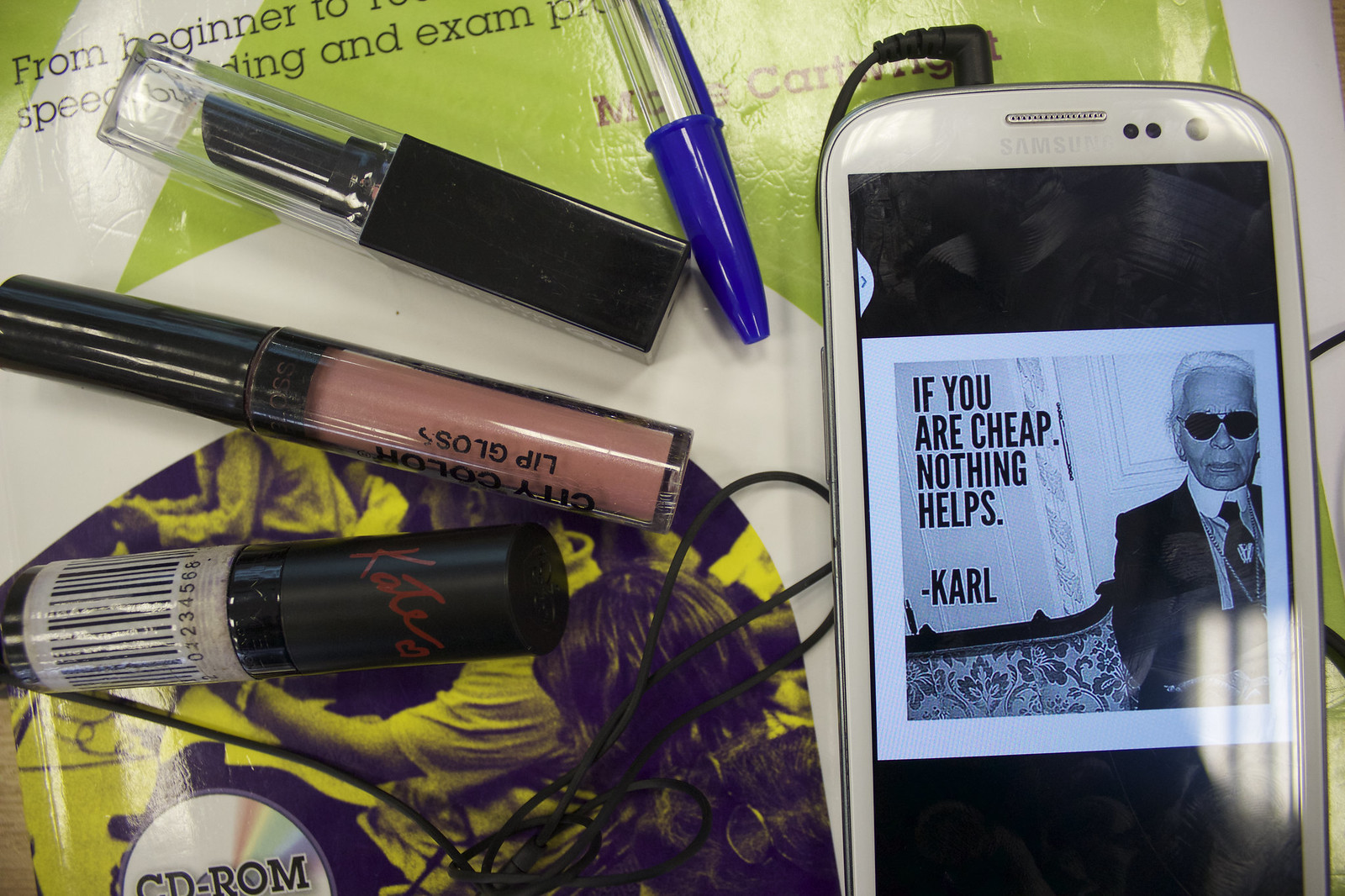The image features an assortment of items arranged on a surface, with a smartphone prominently displayed on the right side. The phone, which has a white outline and appears to be a Samsung model, displays a black-and-white image of an older man with white hair, dark sunglasses, a black jacket, a black tie, and a suit with a white collar. The shirt he is wearing looks speckled. To the left of this image, in bold black lettering, is the quote: "If you are cheap, nothing helps," followed by a dash and the name "Carl." The phone has two small black dots and a slightly larger gray dot in the upper right corner and appears to be plugged into earphones or a charger.

To the left of the smartphone, there is a blue-capped pen at the top, followed by a clear-capped black lipstick bottle, a lipstick with a black top and peach bottom labeled "lip gloss," and another black-cased container with a scanning bar at the bottom. The background features a green and white magazine, book, or flyer with some unreadable black text at the top and a yellow and black image. At the very bottom, there's a partially visible CD labeled "CD-ROM.”